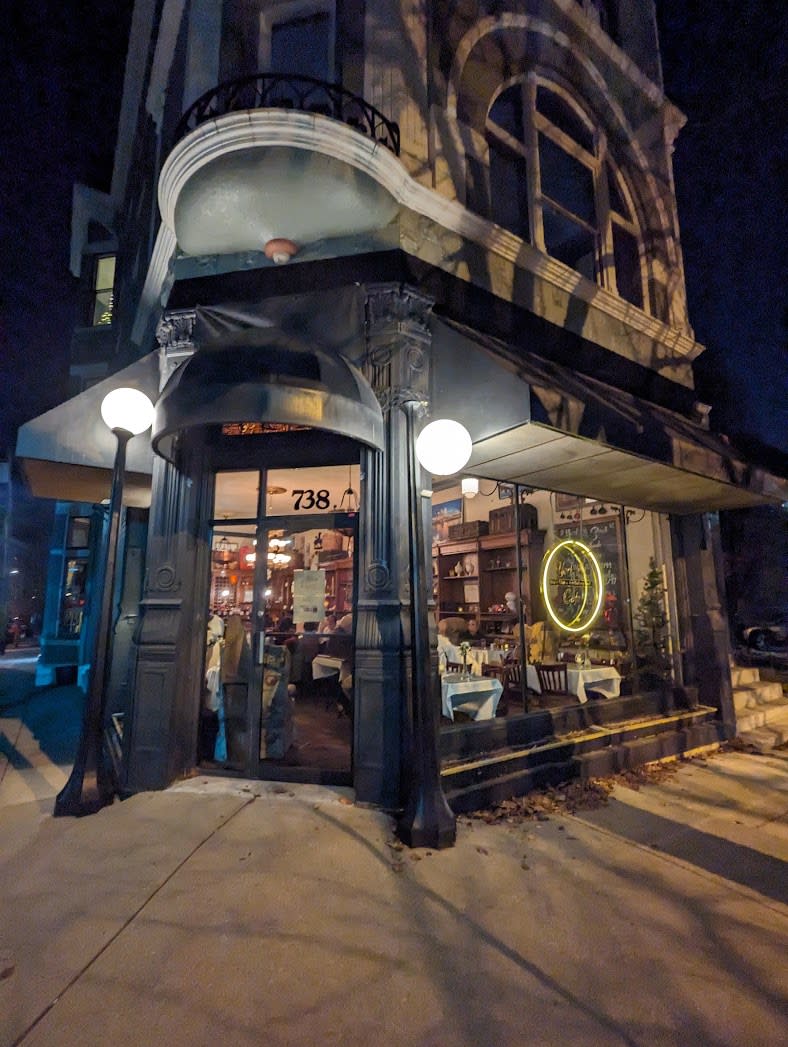The photograph captures a multi-storey corner building with the number 738 prominently displayed above the entrance. The building appears to function as a restaurant or diner, given the visible white tablecloths and black wooden chairs inside. There is a black canopy at the front entrance, resembling an umbrella, and black pillars around it. Flanking the entrance are two floor lamps with spherical orbs that emit a bright white light, attached to black poles. The top part of the building features an arch window and a balcony with black railings, outlined in white trim. The surroundings include a curved sidewalk, gray steps, and a silver or gold car parked nearby. The exterior of the building is predominantly gray with shadows accentuating its architectural details. Notably, the facade has additional black and white awnings on the sides. There are also leaves scattered on the sidewalk adjacent to the building.